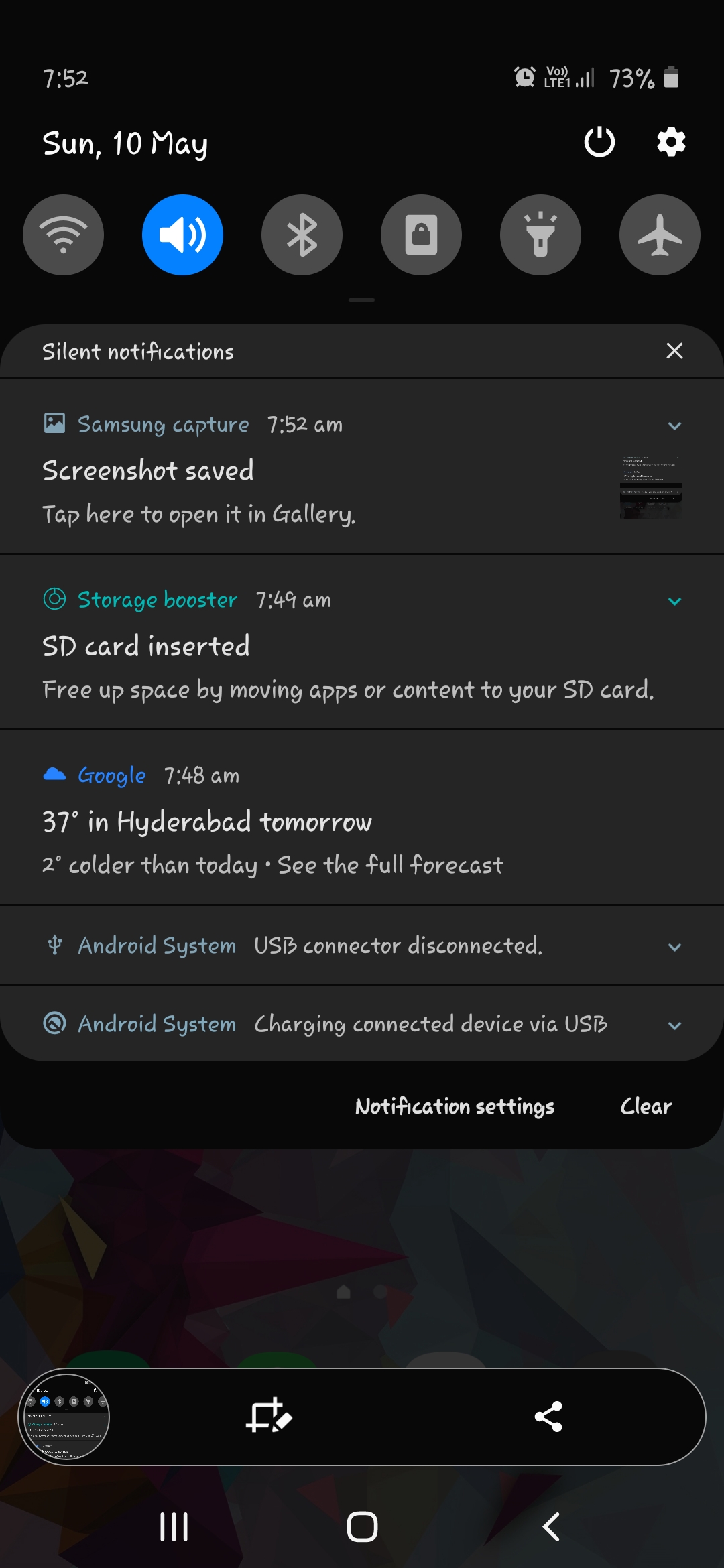Screenshot displaying a smartphone notification panel with numerous details:

- **Top left corner**: The number "7:52".
- **Top right corner**: The word "VoLTE" in white, a white clock icon, and a battery icon displaying "73%".
- **Top**: The date and day reading "Sun, 10 May".

**Notification bar details**:
- **Six circles for quick settings**:
  - First circle: Dark gray with a gray volume icon.
  - Second circle: Blue with a white bell icon and sound waves.
  - Next four circles: Dark gray with icons representing various functions, including a ribbon, light gray square with a dark lock, flashlight, airplane mode, and possibly a screenshot function.

**Silent notifications section**:
- **Notification**: "Samsung capture"
  - Time: "7:52 a.m."
  - Description: "Screenshot saved, tap here to open it in the gallery."
  - Icon: A little square with an image symbol (sun and mountains).

**Additional notifications**:
- **Green header**: "Storage booster"
  - Time: "7:49 a.m."
  - Action: SD card inserted, suggesting freeing up space by moving apps or content. 

- **Blue header**: "Google"
  - Time: "7:48 a.m."
  - Weather update: "37 degrees, height or bad tomorrow, two degrees colder than today, see the full forecast."

- **Android system notifications**:
  - First entry: "USB connector disconnected" with a down arrow.
  - Second entry: "Charging connected device via USB" with a down arrow preempted by two fine black lines. 

**Bottom banner and controls**:
- **Mutely colored background**, possibly a screensaver with shades of gray and burgundy.
- **Black banner at bottom**:
  - Thumbnails: Screenshot of the current page, a half square with a white pencil, and a white search icon.
  - Navigation buttons: Three white bars (menu), a back button, a square (recent apps), and an arrow pointing left.

This cleaned-up caption ensures clarity and provides a detailed description of the visual elements and respective functions within the screenshot.